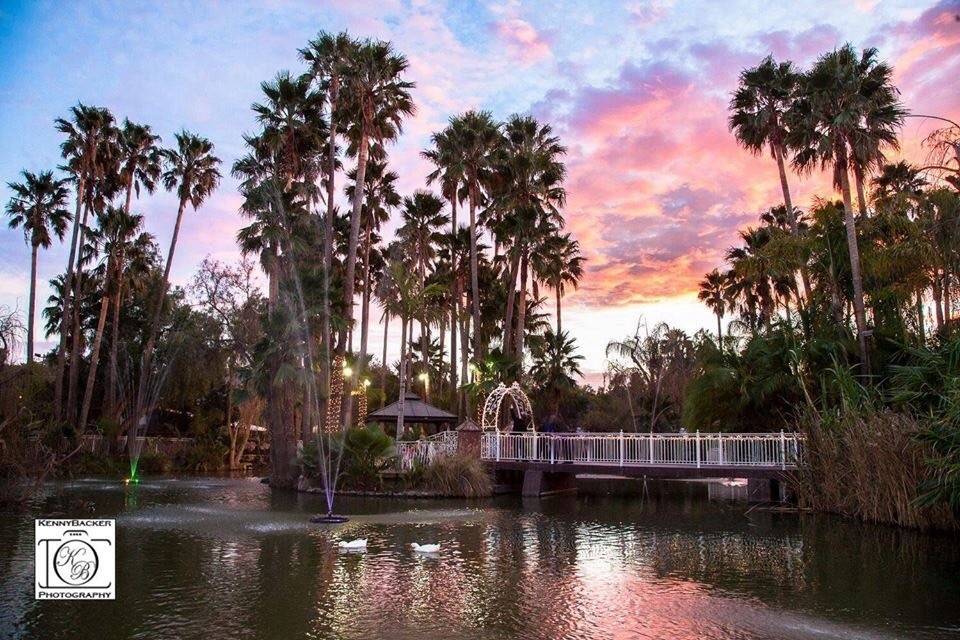The image captures a vibrant tropical water attraction set during a picturesque sunset, with hues of pink, orange, purple, and blue coloring the sky. Tall palm trees surround the scene, adding to the lush, exotic ambiance. At the center, a body of water features fountains gracefully spraying, and ducks can be seen floating on the serene surface. 

A white wrought iron bridge with vertical spindles spans across the water, leading to a tiny island. This bridge, which includes a canopy entrance, is topped with a wrought iron arbor near the island. Beyond the island, a quaint tiki hut can be seen, adding to the idyllic setting. 

Further in the background, there's another island without a visible bridge, enhancing the sense of exploration and mystery. There is also an edge of a landmass on the right, adorned with greenery. The bottom left of the image credits "Kenny Backer Photography" with a camera icon. The overall scene suggests a location within a resort or hotel, offering a serene and appealing destination for visitors.